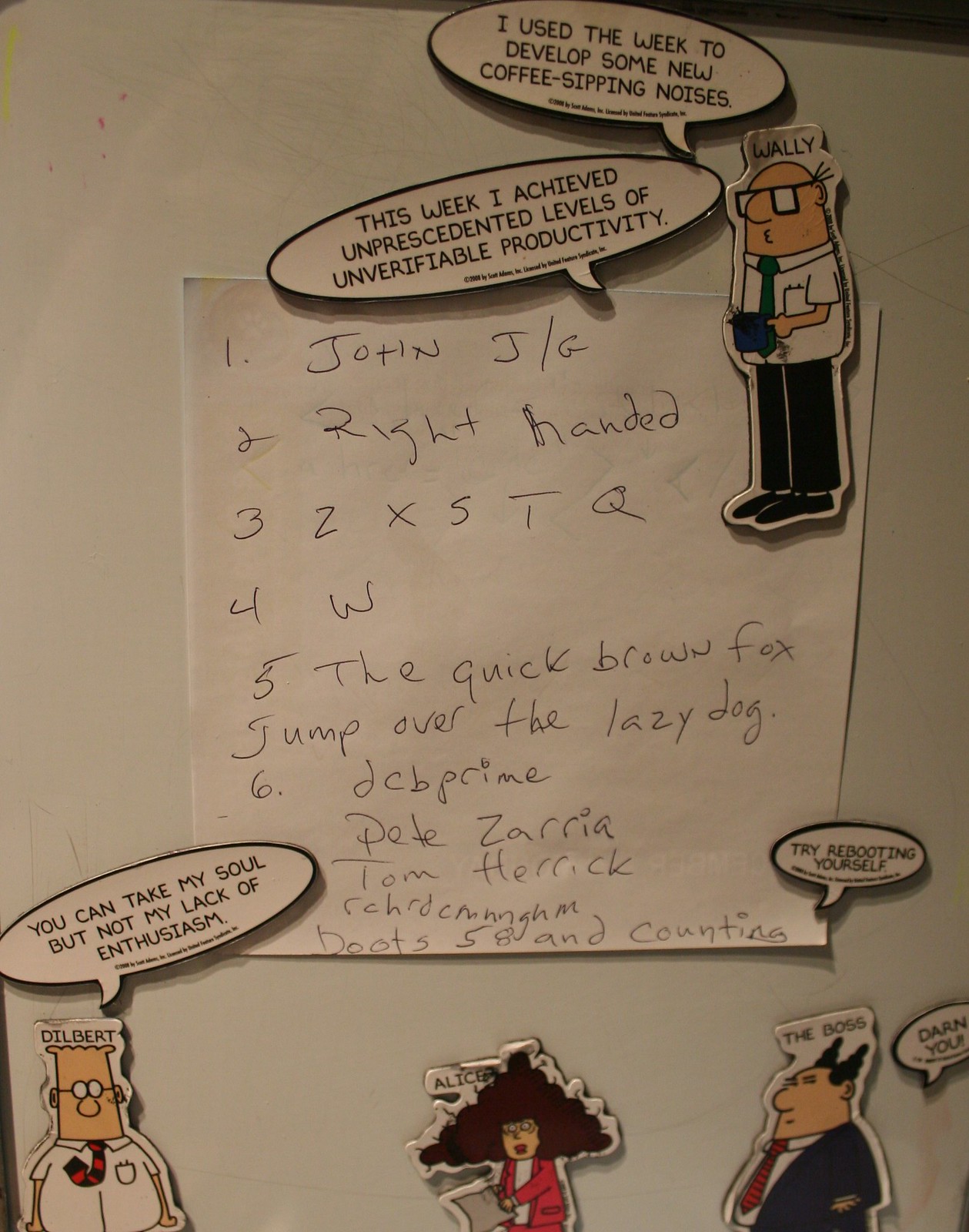This image showcases a magnetic refrigerator surface, crowded with quirky magnets featuring characters from the Dilbert comic strip, including Wally, Dilbert, Alice, and the Boss. Surrounding these characters are numerous comic-style quote bubbles with amusing phrases such as "I used the week to develop some new coffee-sipping noises," "This week I achieved unprecedented levels of unverifiable productivity," "You can take my soul but not my lack of enthusiasm," and "Try rebooting yourself, darn you." Centrally taped to the refrigerator is a handwritten list that includes the following: 1. John J/G, 2. Right-handed, 3. ZXSTQ, 4. W, 5. The quick brown fox jumps over the lazy dog, 6. DCB prime, Pete Zaria, Tom Herrick, RCHRD, CN, NNGHM, Boots, 58 and counting. The arrangement creates an eclectic mix of humor and casual notes, capturing a playful work environment atmosphere.